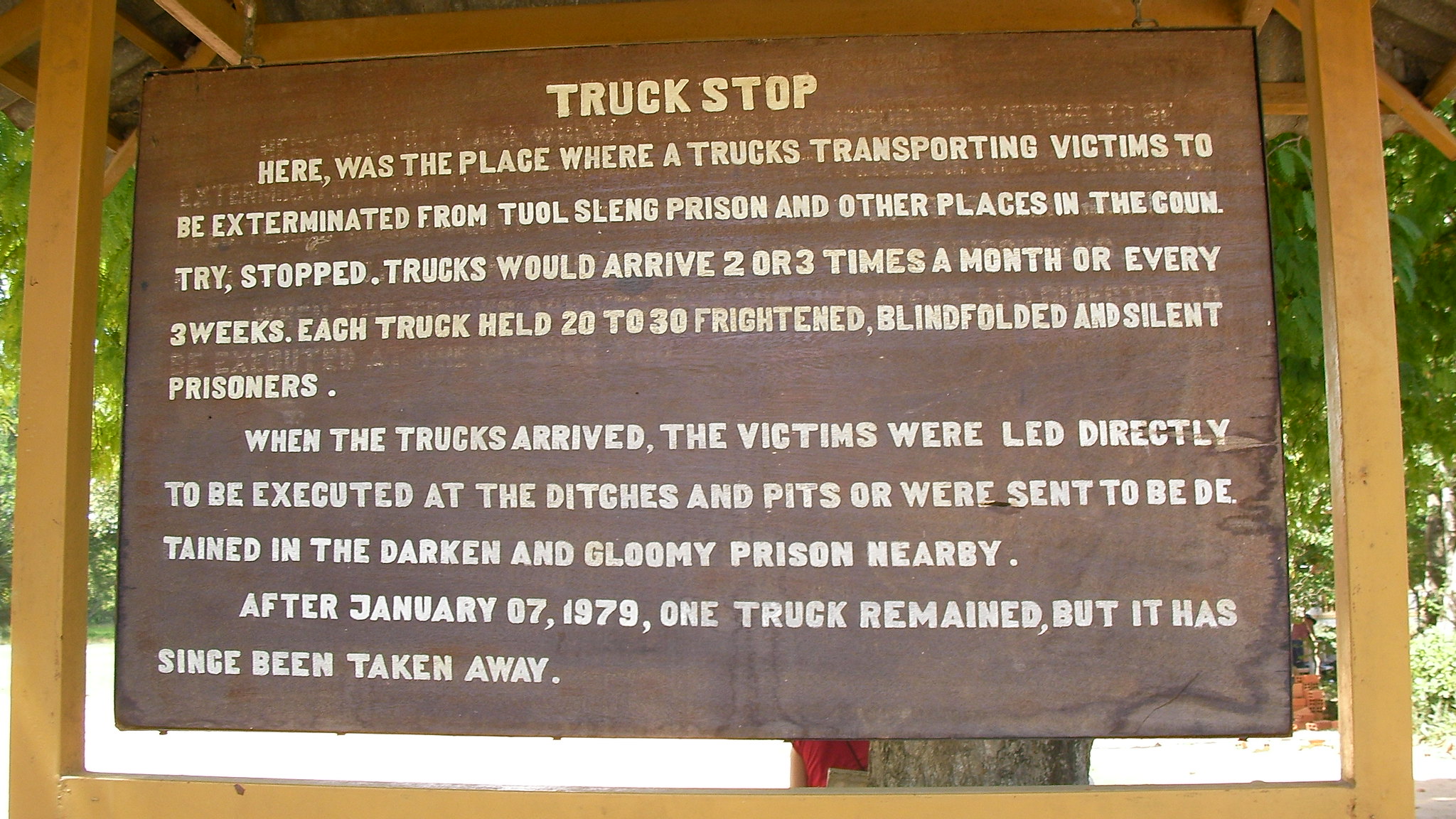The image depicts a full-color photograph taken outdoors during the daytime, showcasing a prominent brown wooden sign adorned with white lettering. This sign, which reads "Truck Stop," is sheltered under a roofed wooden structure, providing protection from the rain. The photograph captures a serene natural setting, surrounded by several green-leaved trees on both the left and right sides. 

In the background, subtly situated in the lower right-hand corner, a person can be discerned upon careful examination. The sign’s text elaborates on a grim historical context: it marks the spot where trucks, carrying frightened, blindfolded, and silent prisoners from Tuol Sleng Prison and other locations, arrived every two to three weeks. These prisoners were then led either to immediate execution at nearby ditches and pits or detained in a dark, gloomy prison. A poignant note mentions that after January 7, 1979, one truck remained, but it has since been removed.